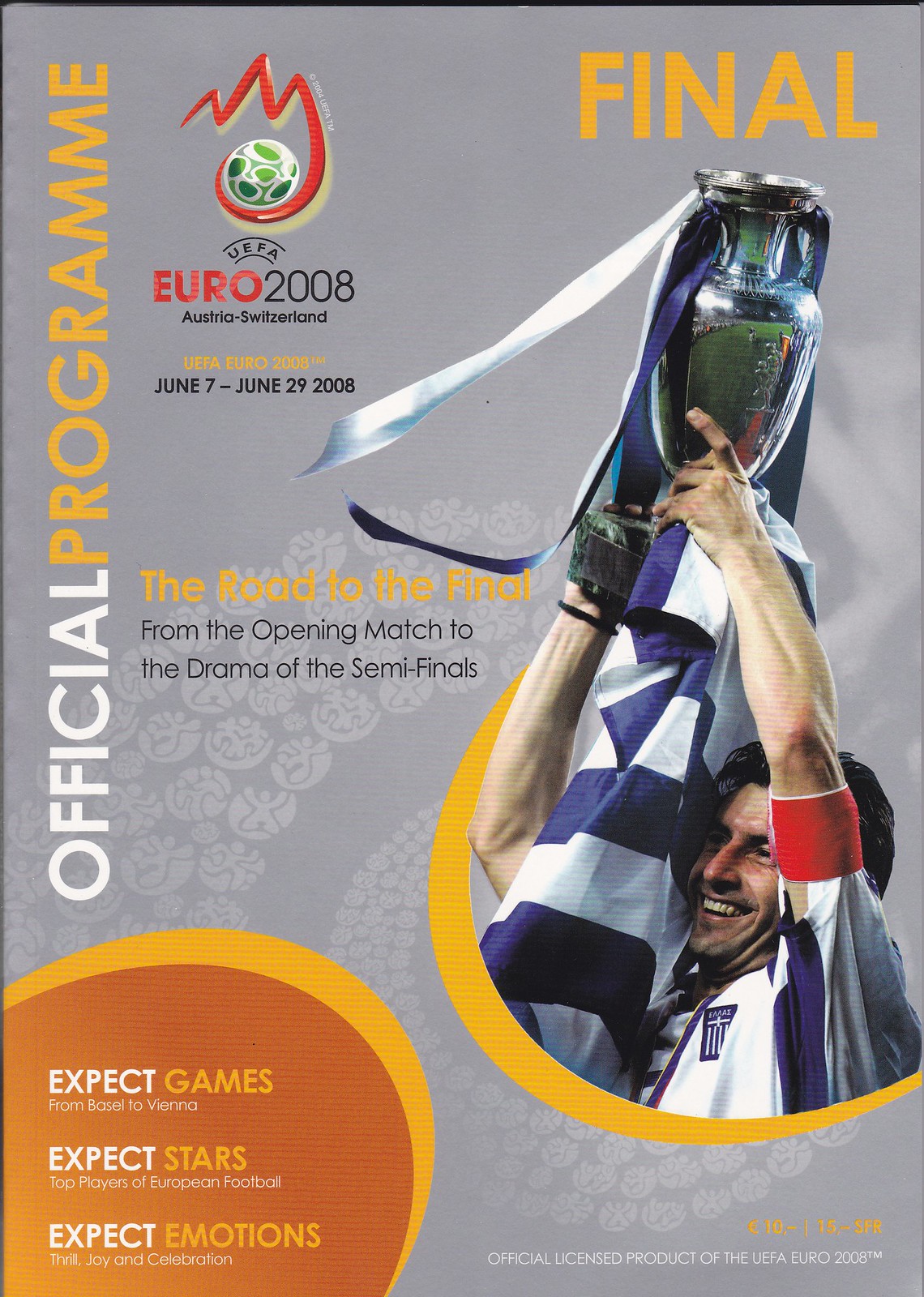This is an image of the cover of an official program for the UEFA Euro 2008 held in Austria and Switzerland from June 7 to June 29, 2008. The cover is in portrait view with a gray and yellow-orange background. The top right corner prominently features the word "Final" in yellow. Just below, there is a red, green, and white logo depicting a flame holding a soccer ball, with text reading, "UEFA Euro 2008 Austria Switzerland." More detailed text below states the event dates, June 7 to June 29, 2008.

Along the left side of the cover, the words "Official Program" are displayed vertically, with "Official" in white and "Program" in yellow. The center of the cover showcases a jubilant soccer player wearing a white jersey with red accents, holding a silver trophy adorned with blue and white sashes. The player also holds a blue and white striped flag, and his beaming smile captures the celebratory spirit of the event.

Beneath the player's image, the text reads, "The road to the final: From the opening match to the drama of the semifinals," in yellow and black. The bottom left corner highlights the anticipation for the event with phrases in yellow and orange, saying, "Expect games from Basel to Vienna. Expect stars from top players of European football. Expect emotions of thrill, joy, and celebration." The bottom right corner confirms the authenticity of this program, indicating it as an "Official Licensed Product of the UEFA Euro 2008."